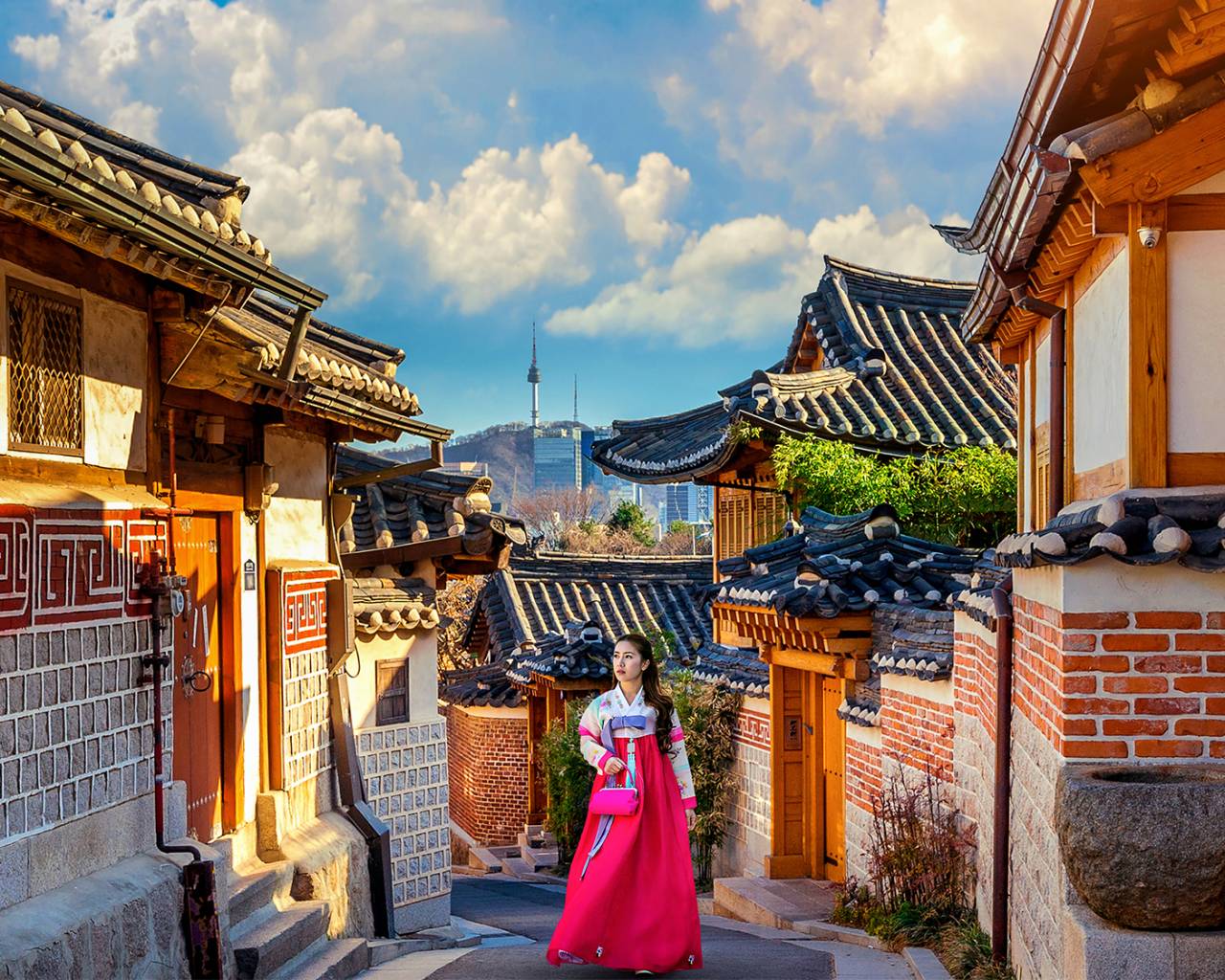This is an outdoor daytime photograph or painting set in a traditional Asian city, suggested to be either Japanese or Chinese. The scene features a narrow, paved street lined with colorful buildings that showcase traditional Asian architecture, notable for their curvy, pointed, pagoda-style roofs. The buildings, made of wood or brick in varied hues including brown, gray, burgundy, and blue, are complemented by ornamental bushes and small rooftop gardens. The street, exclusively for pedestrians, ascends slightly and winds through the tightly packed homes.

In the center of the photograph stands a young Asian woman in her 20s, dressed in a traditional outfit. She has long dark brown or black hair cascading over her shoulder and wears a flowing dress—the top part is white with long sleeves, adorned with hot pink and possibly turquoise accents, while the skirt is a vivid pink that reaches the ground. A purple bow with a long ribbon decorates her waist, and she carries a pink purse with a snap closure in her right hand. Her serene expression suggests she is either posing or admiring the surrounding architecture, as she gazes upward to the left.

The background reveals a clear, bright blue sky with scattered white clouds. In the distance, there's a tall hill or small mountain crowned by a tower resembling an observation platform or revolving restaurant. The city skyline at the base of the hill features several skyscrapers tucked into the landscape, further emphasizing the blend of traditional and modern elements in this picturesque setting.